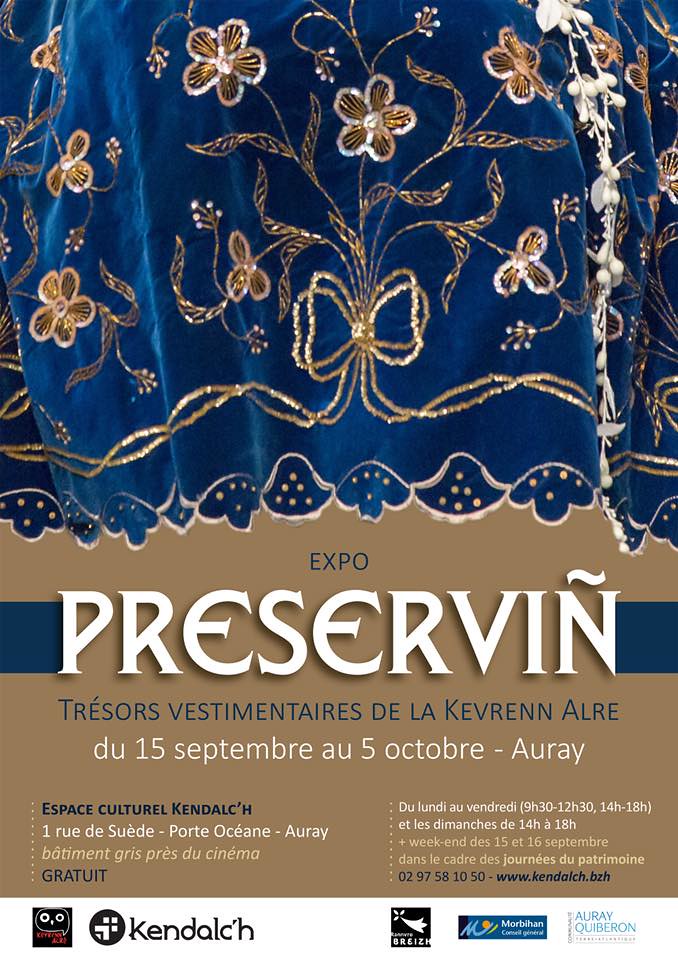This advertisement poster promotes the "Expo Préservin: Trésors Vestimentaires de la Caverne Alleray," taking place from September 15th to October 5th. The top half of the poster features a piece of blue felt intricately embroidered with gold flowers and flower stalks, adding a luxurious and artistic detail to the design. The bottom half of the poster is tan or light brown and contains multiple lines of white and dark blue text. Details included on this section are the event's dates, location "Alleray, Espaces Culturelles Kandalks," specific location information "One Rue du Suede, Porte Ocean Alleray," and additional notes such as "Batamante Grise Presse du Cinéma Gratuit," available from Monday to Friday, 6:30 to 9:00 AM. The overall design is visually balanced with the floral print situated on the top half and the textual information on the bottom half, making it an eye-catching promotional piece. The poster also includes a phone number, "029-758-1050," and a website, "www.kendalch.bzh," for further inquiries.